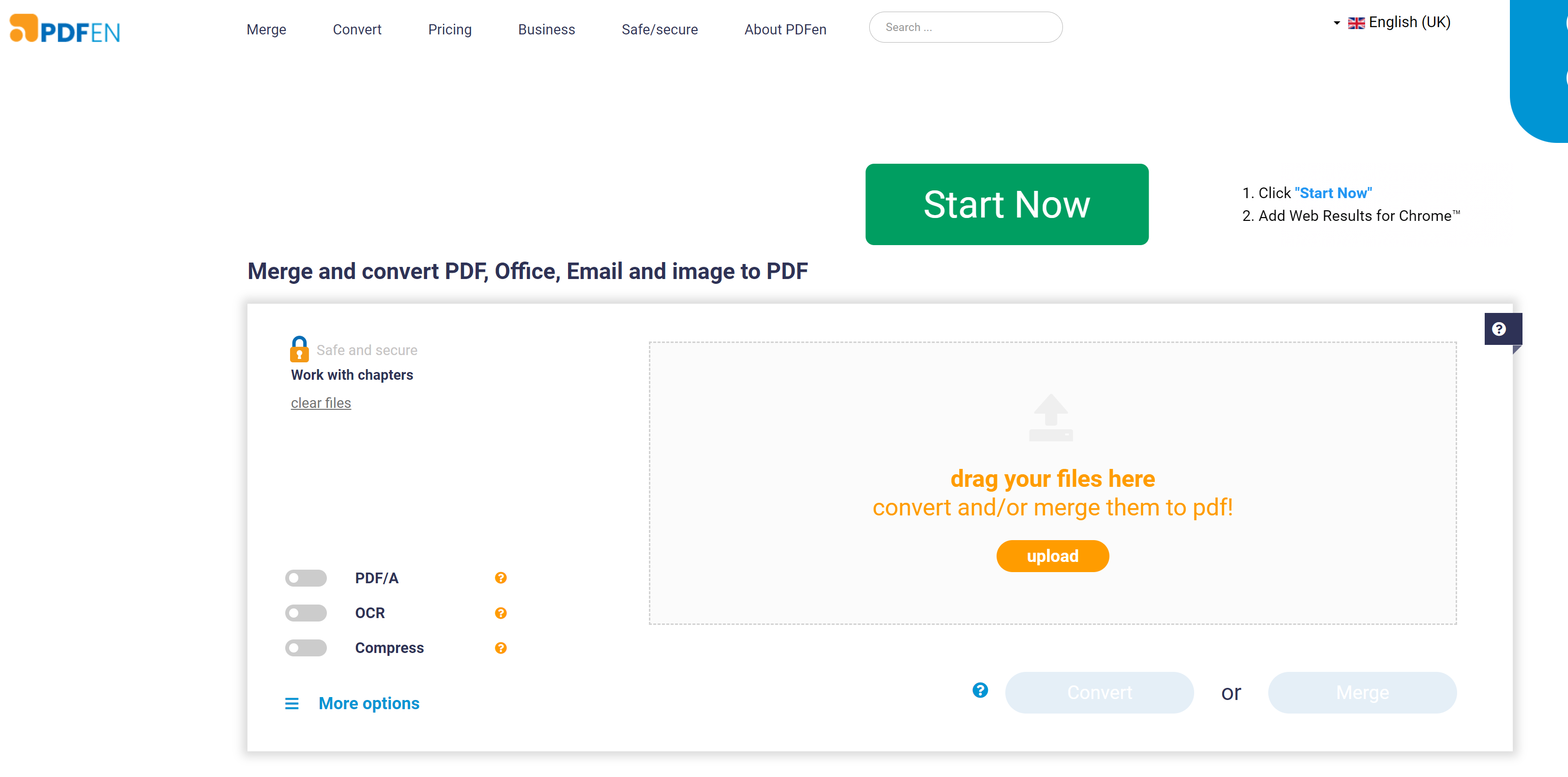**Descriptive Caption:**

The image is a screenshot of a website with a clean white background. Prominently positioned at the top left corner is the text "PDF EN," where "PDF" is styled in bold blue font and "EN" in a lighter, thinner blue. Adjacent to this text is a distinct logo composed of two orange elements: a circle in the bottom left and a boomerang shape extending upward and to the right from the circle.

To the right of the logo, medium-gray navigation text spans from left to right, listing the following options: "Merge," "Convert," "Pricing," "Business," "Safe/Secure," and "About PDF EN." Further right, there is a search box containing placeholder text that reads "Search..." Next to the search box, a Union Jack flag indicates the language setting, flanked by gray text labeled "English (UK)" with arrows to the left and right suggesting a dropdown menu.

Beneath this header is the main body of the website. A prominent green button with rounded corners and bold white text invites visitors to "Start Now." To the right of the green button are two textual lines: the first, in blue, reads "'One click start now,'" while the second line, in medium gray, states "Add web results for Chrome."

A white pop-up occupies the central space, featuring a heading: "Merge and convert PDF, office, email, and image to PDF." Inside this pop-up, an orange lock icon with a blue loop appears on the top left, next to light gray text declaring "Safe and secure." Beneath this, bold text reads "Work with chapters," and further down, medium-gray underlined text states "Clear files."

Positioned to the right within the pop-up, a light gray box prominently displays orange text instructing users to "Drag your files here, convert and/or merge them to PDF." The final element at the bottom of the pop-up is an orange button with white text that says "Upload." 

This comprehensive layout offers a clear and user-friendly interface for PDF management tasks, underscoring ease of use and security.